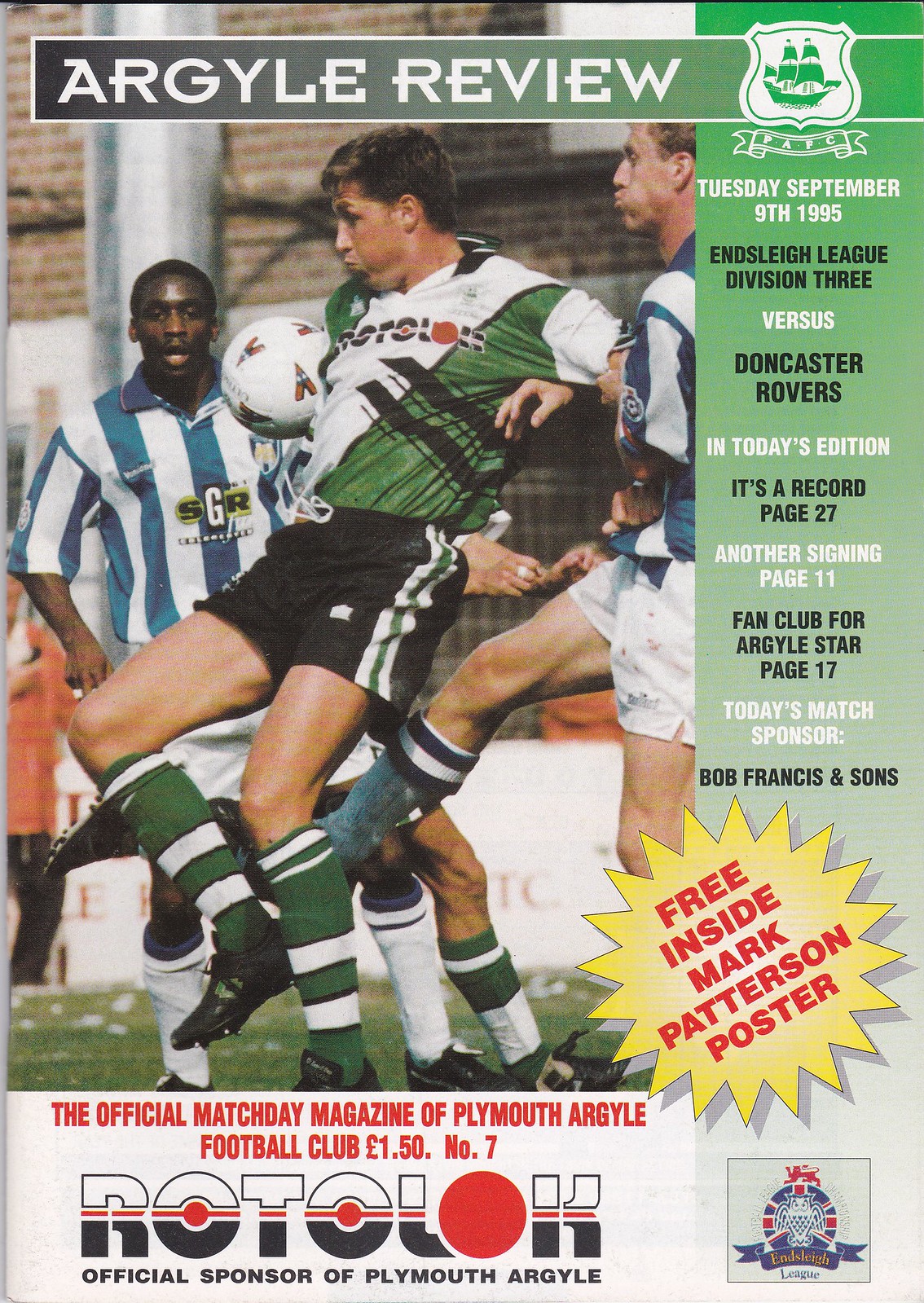This is a color photograph of the cover of an old football program titled "Argyle Review." The scene features an Argyle player in a green and white jersey with black shorts and green socks, kneeing a soccer ball into the air while flanked by two opposing players in blue and white vertically striped jerseys and white shin guards. The background showcases a brick wall, framing the athletes in action. The program is dated Thursday, September 9th, 1995, and prominently states, "Ensley League Division III vs. Doncaster Rovers." In a green strip on the right, it mentions features from today's edition including "It's a Record, page 27," "Another Signing, page 11," and "Fan Club for Argyle Star, page 17." At the bottom right, a seal proclaims "Free Inside Mark Patterson Poster," written diagonally. Below the image, the text reads "The Official Match Day Magazine of Plymouth Argyle Football Club," priced at one pound fifty. It also notes the official sponsor as Rotoloc, and identifies this as issue number 7. Additionally, today's match sponsor is listed as Bob Francis and Sons.